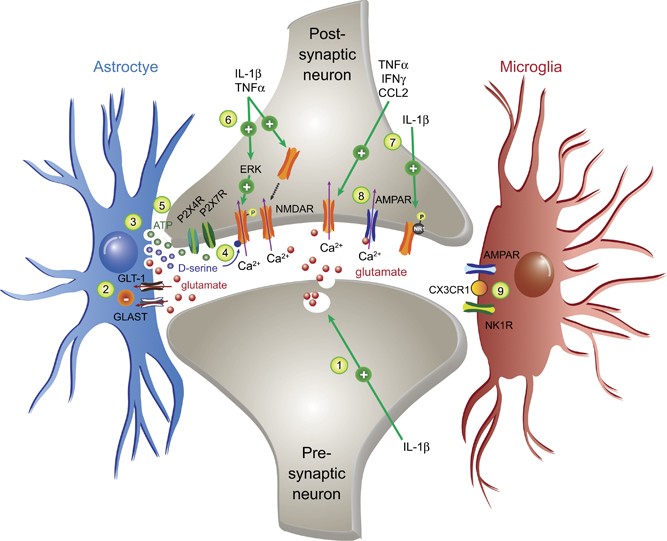This intricate scientific diagram illustrates the nerve systems with detailed scientific terminology and abbreviations. At the core, there are two prominent gray shapes; the upper one is labeled as the postsynaptic neuron, while the lower one, resembling a rounded-off Y or a pelvis bone attached to a spine, is labeled as the presynaptic neuron. On the left side, a blue spindly structure is identified as an astrocyte, and on the right, a red spindly structure labeled microglia. The diagram features numerous smaller illustrations and symbols in green, orange, and blue, indicating various scientific processes and molecules. Green arrows point to different parts of the diagram, and scattered red dots further detail the composition and function of these nerve systems. The image is densely packed with both labeled and unlabeled elements, emphasizing its complex and scientifically specific nature.